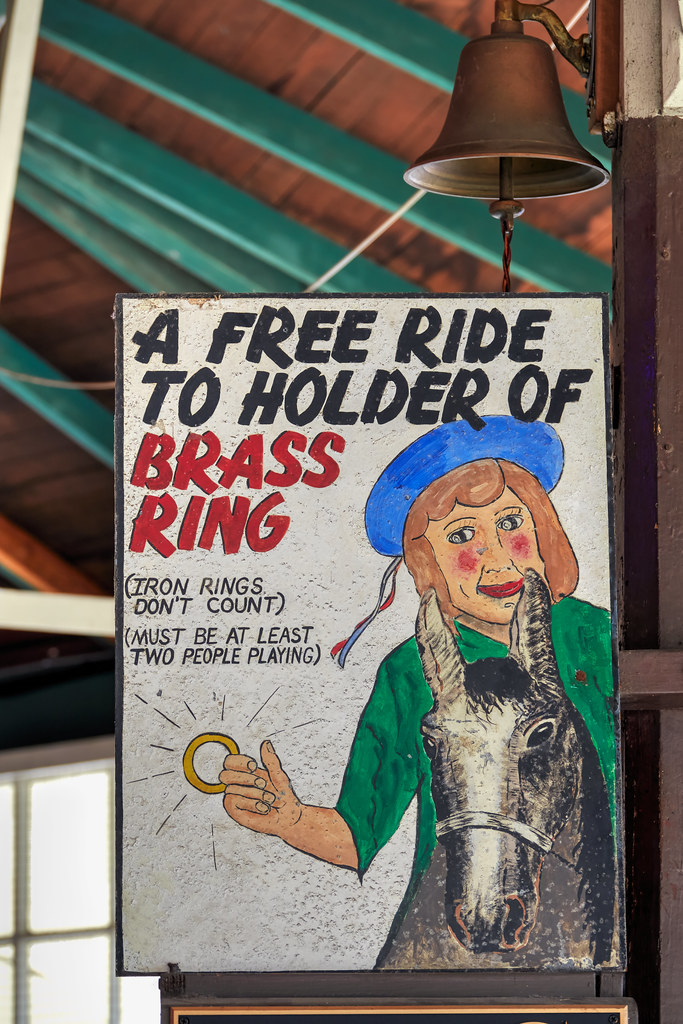The image features an old, rectangular wooden sign with a white background and black edging. At the top of the sign, bold black text reads "A Free Ride to Holder of Brass Ring," with the words "Brass Ring" highlighted in red. Below this, additional text in black states, "Iron rings don't count," and "Must be at least two people playing." 

Accompanying this text is a detailed drawing of a woman with brown hair, wearing a green shirt and a blue hat adorned with red, white, and blue tassels. She holds a large, golden-colored ring in her right hand. The woman is seated on a gray horse, of which mainly the head is visible, featuring white markings on its nose.

The sign is set against a rustic background with elements suggesting it is hung outside a building. Above the sign, a prominent brown metal bell with a string attached hangs from the brown, wood-paneled ceiling, which is supported by lighter green beams. To the left of the sign, there is a window through which light filters in, adding to the rustic charm of the setting.